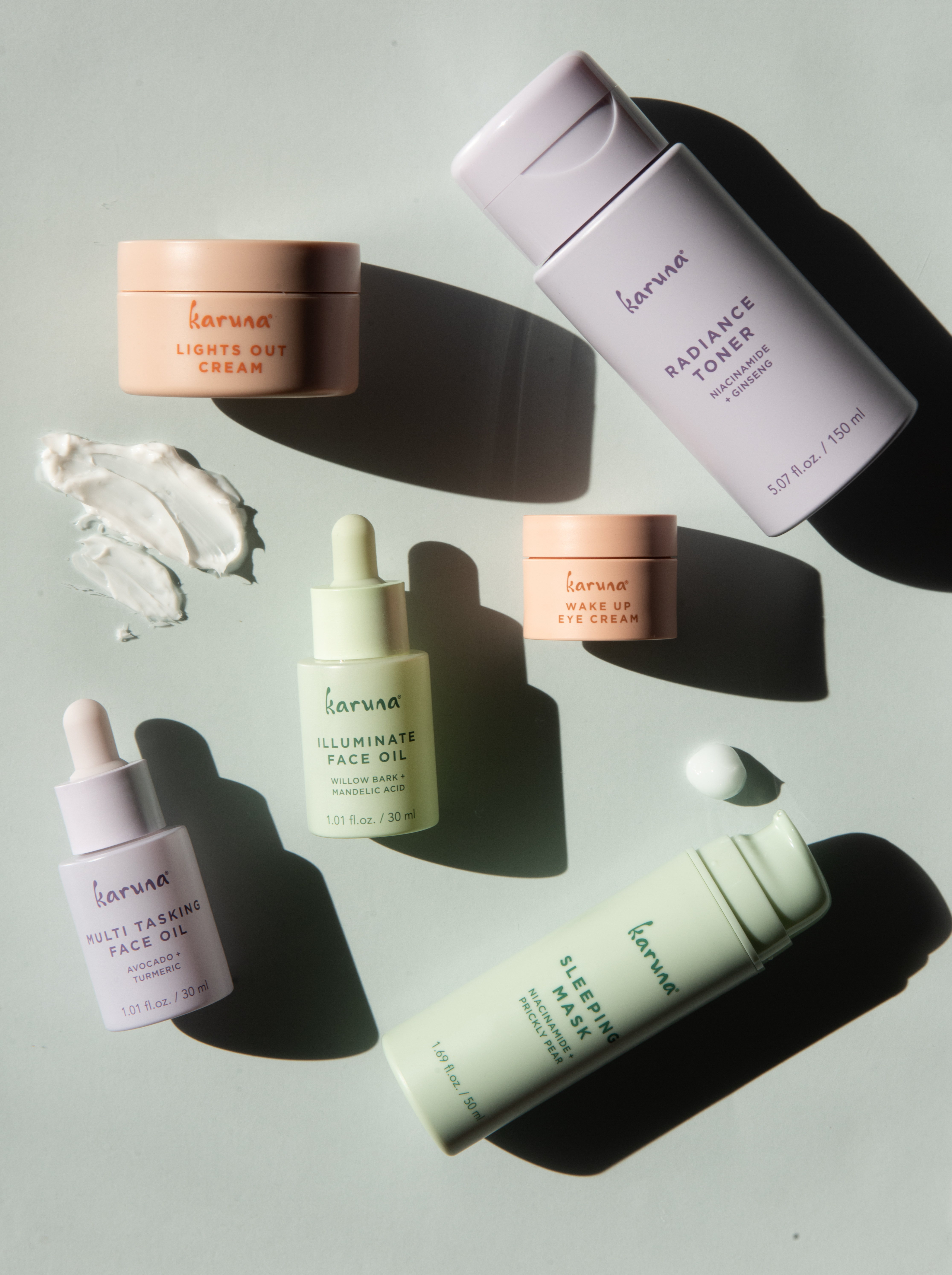In the image, there's a neatly arranged display of various skincare products set against a light green background. Starting from the top right, there is a white bottle labeled "Caruna Radiance Toner" containing 5.7 fluid ounces. To its left, there's a round, peach-colored jar labeled "Caruna Lights Out Cream," with some of the cream smeared on the backdrop beside it. Below that jar, another product labeled "Caruna Illuminate Face Oil" is placed in a whitish-green dropper bottle featuring willow bark and mandelic acid, holding 1.01 fluid ounces or 30 milliliters.

Adjacent to this, there is a smaller, peach-colored jar marked "Caruna Wake Up Eye Cream." To the far left, a white bottle labeled "Caruna Multitasking Face Oil with Avocado and Turmeric" comes in a dropper bottle, also containing 1.01 fluid ounces or 30 milliliters. Finally, in the lower left corner, a light green bottle is labeled "Caruna Sleeping Mask with Niacinamide and Prickly Pear," with a dab of white cream near its tip.

Each product casts strong shadows, indicating distinct and direct lighting. The pastel-colored packaging of all products suggests they are potentially marketed for an online retail store.